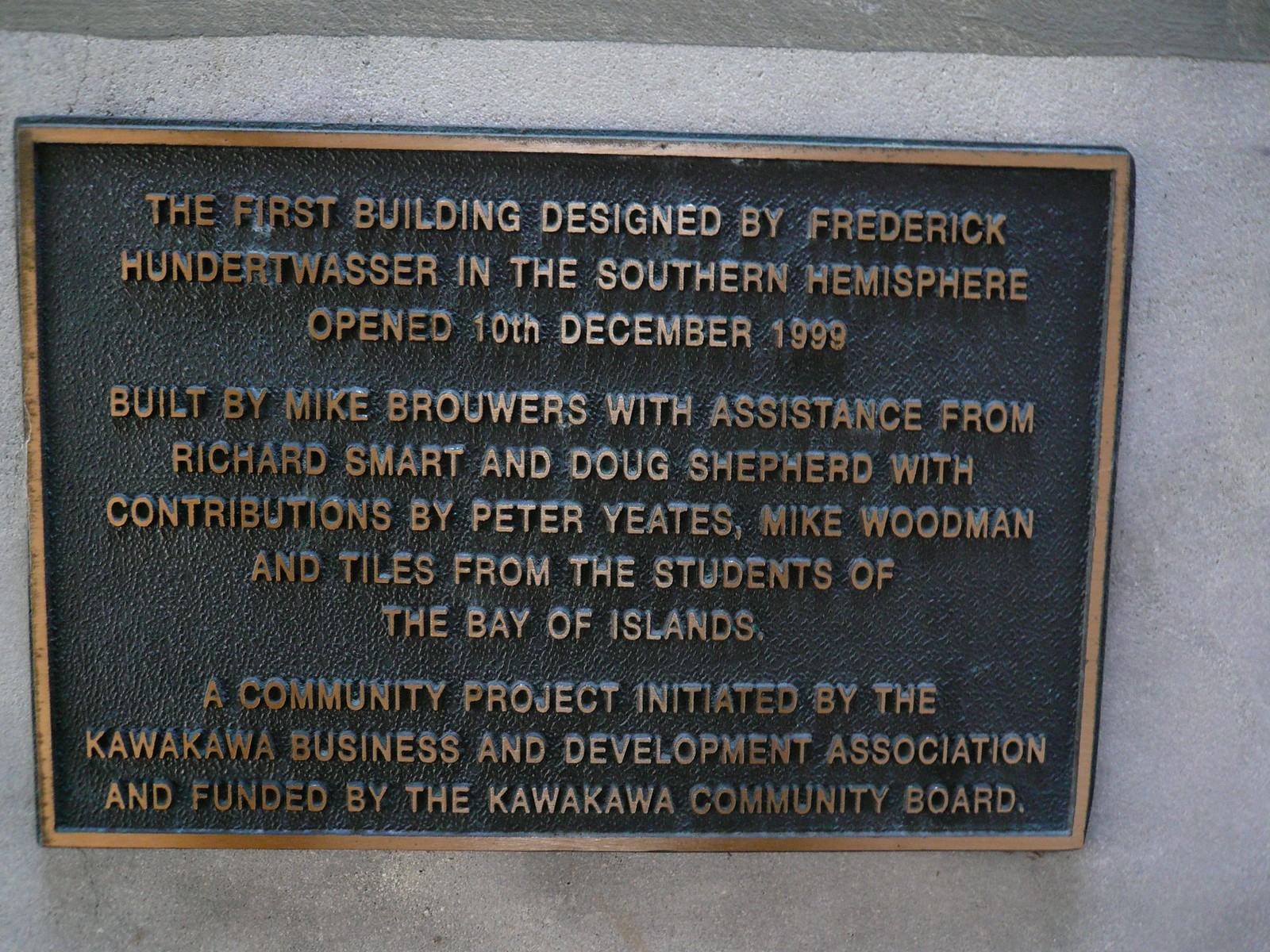The image showcases a well-crafted plaque mounted on a gray stone wall. The plaque, centered in the frame and seemingly positioned outdoors on a historical building, exudes a timeless elegance with its black background, raised black text, and an off-gold, brass-like border that hints at its age while still looking well-maintained. The inscription honors the first building designed by Frederick Hunter Wasser in the Southern Hemisphere, which opened on December 10, 1999. This building was constructed by Mike Browers, with help from Richard Smart and Doug Shepard, and further contributions by Peter Yeats, Mike Woodman, and tile work by the students of the Bay of Islands. This community-driven project was initiated by the Kawakawa Business and Development Association and financed by the Kawakawa Community Board. The plaque's polished yet aged appearance allows the text to stand out sharply, making it easy to read and visually striking against the backdrop of varying shades of gray stone.